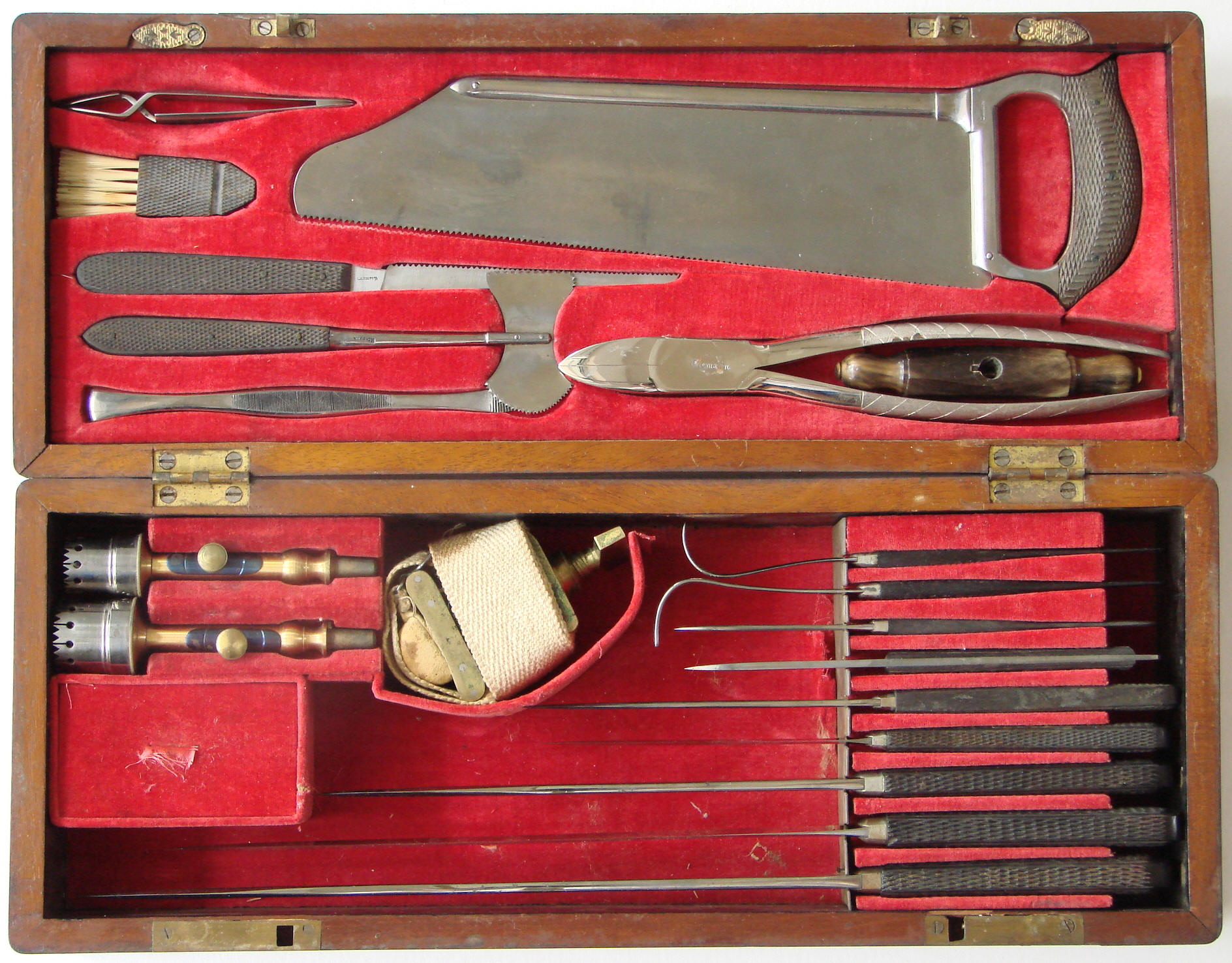This is a photograph of an antique wooden case, opened to reveal a red velvet-lined interior meticulously arranged with a collection of vintage tools, possibly surgical instruments from the 1700s or 1800s. At the top, the case features a variety of sharp instruments including saws, knives, tweezers, and pliers. Notably, each tool has a black handle and rests in its own designated slot within the red velvet, ensuring a neat presentation. The upper section contains saws and sharp cutters, while the lower section holds an assortment of curved and straight, long, pointy instruments. Despite some uncertainty about the exact use of each tool, the presence of meticulous tools like tweezers, a brush, and potential thimbles suggests this could be a historical surgical kit, emphasizing its vintage and professional appearance. The clear photograph captures this intriguing and possibly unsettling set of instruments in striking detail.